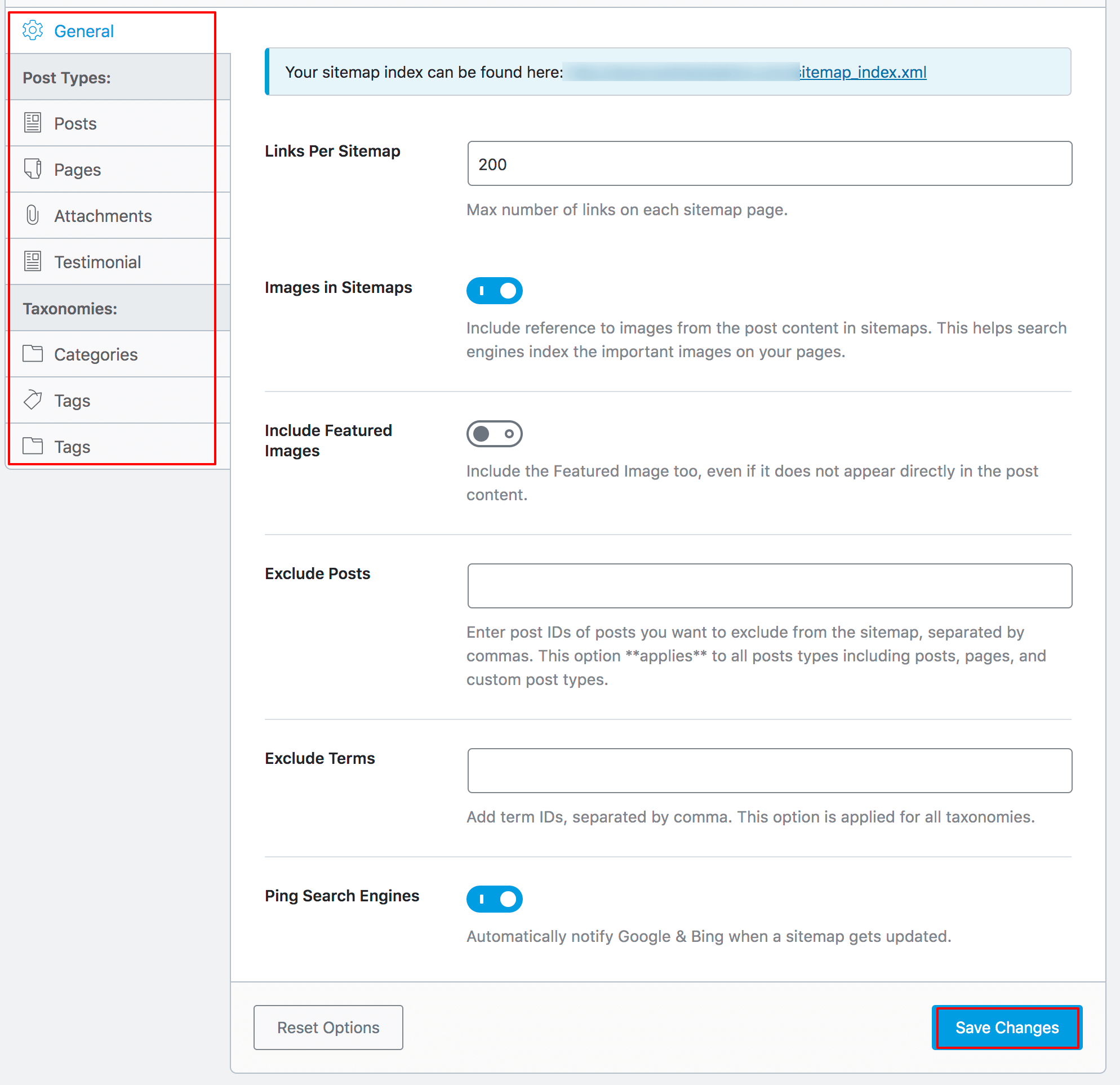The image is a screenshot of an application's or website's settings page. In the upper left-hand corner, there is a red box, likely added post-capture using a photo editing software like Photoshop, to draw attention to a list of categories at the top. The list features a small blue gear icon next to the word "General" in blue font, followed by a section labeled "Post Types" which lists "Posts," "Pages," "Attachments," and "Testimonials." Below that, another section labeled "Taxonomies" lists "Categories" and "Tags."

On the right side of the image, a white background displays various settings. There is a blue banner at the top indicating, "Your sitemap index can be found here:" followed by a blurred-out URL. Below this, several settings are listed:
- "Links per sitemap: 200"
- "Images in sitemap: Turned On"
- "Include featured images: Turned Off"
- "Excluded posts:" followed by a blank text box
- "Excluded terms:" followed by a blank text box
- "Ping search engines:" Activated

In the bottom right-hand corner, another red box highlights the "Save Changes" button, which is blue with white font.